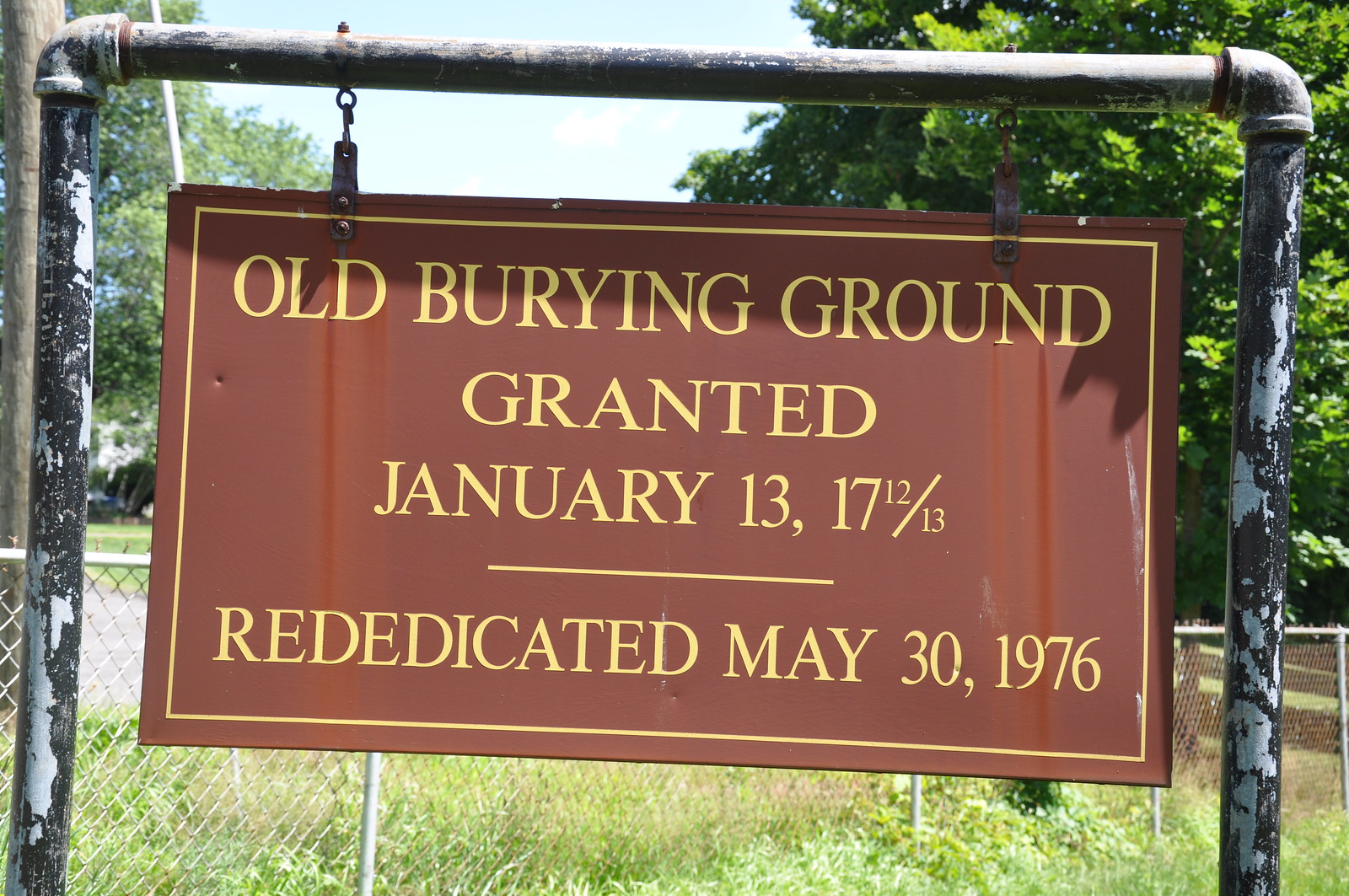The image captures a photograph of a sign situated in what appears to be a cemetery or possibly a burial ground, given the context provided. The sign reads, "Old Burying Ground, granted January 13, 1712/13, rededicated May 30, 1976." It hangs from two poles that resemble pipes. These poles are worn, chipped, and exhibit a multicolored appearance, likely due to aging. Behind the sign, a fence is visible along with a backdrop of trees and grass, suggesting a natural, possibly park-like setting. The day appears bright, enhancing the details of the scene.